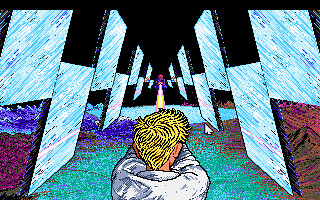The image showcases a detailed piece of artwork, likely in the style of pixel art, potentially from a video game. Dominating the lower part of the image is a person with short, blonde hair and a white shirt, viewed from the back. The figure appears to be engaged in an action, possibly shooting, as a distinct orange beam extends from their position towards a distant purple object. The setting resembles a futuristic or otherworldly environment, with a dark black skyline above and a multicolored floor below, transitioning from light blue in the back to purple, red, and teal towards the front, where the individual stands. The scene is flanked by rectangular panels, reminiscent of glass or mirrors, forming a symmetrical corridor that enhances the depth and geometric complexity of the space.